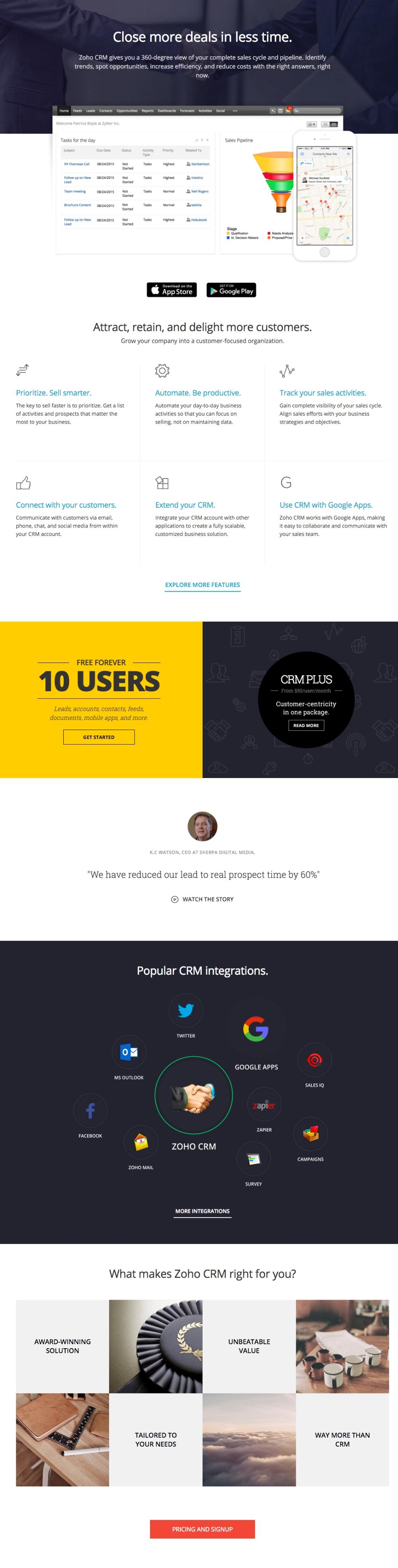In this image, which appears to be a screenshot of a promotional website, the central focus is a headline written in white text that reads, "Close More Deals in Less Time." This headline is set against a background image of two individuals wearing suits and shaking hands, emphasizing the theme of business success and partnership.

Below the headline, there is a section that seems to be a graphical area, although the small size and resolution make it difficult to discern specific details. On the right side of this graphical element is an inverted bottle icon displaying multiple colors: orange, green, red, and yellow.

Further down, two rectangular buttons provide options to download an app, with the left button showing the Apple Store logo and the right button featuring the Google Play logo.

Beneath these buttons, the text reads, "Attract, Retain, and Delight More Customers," indicating the core objectives of the service being advertised. This message is followed by a series of six sections arranged in two rows:

- Top Row:
  - "Prioritize: Set Smarter"
  - "Automate: Be Productive"
  - "Track Your Sale Activities"

- Bottom Row:
  - "Connect with Your Customers"
  - "Send Your CRM"
  - "Use CRM with Google Apps"

At the very bottom of the image, there are multiple small images depicting various scenes, including the sky and tables, likely serving as placeholders or supplementary visual elements.